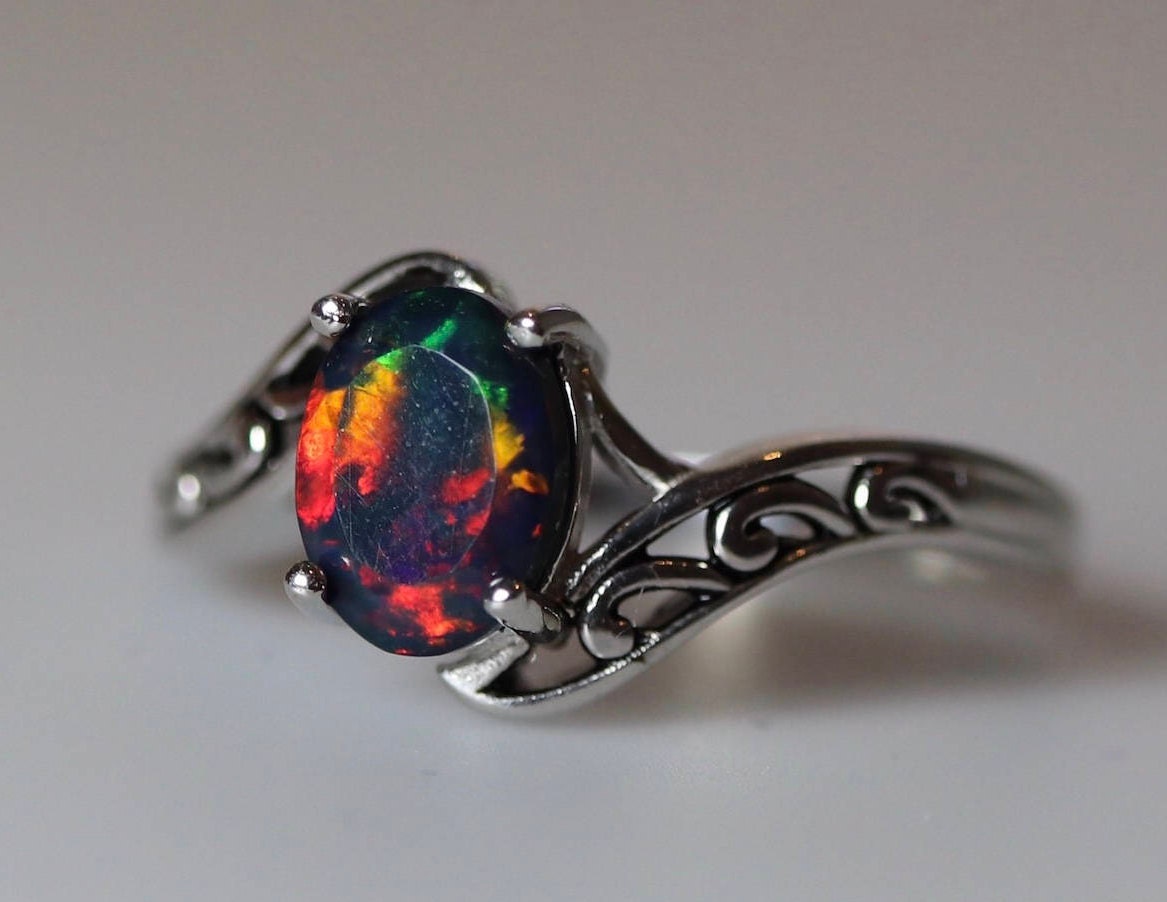This close-up image features a silver ring centered against a plain white background. The focal point of the ring is an oval gemstone, likely a black fire opal, which displays an array of iridescent colors including red, orange, yellow, green, and purple. The majority of the gem appears black, with bright flecks of color distributed across its surface—green near the top, yellow towards the center, and red and orange towards the bottom. The ring's band showcases an intricate, wavy design reminiscent of ocean waves, providing an elegant frame for the vibrant gemstone. The shadow of the ring can be seen in the bottom right of the image, and the depth of field is shallow, leaving the background and parts of the ring out of focus and slightly blurred.